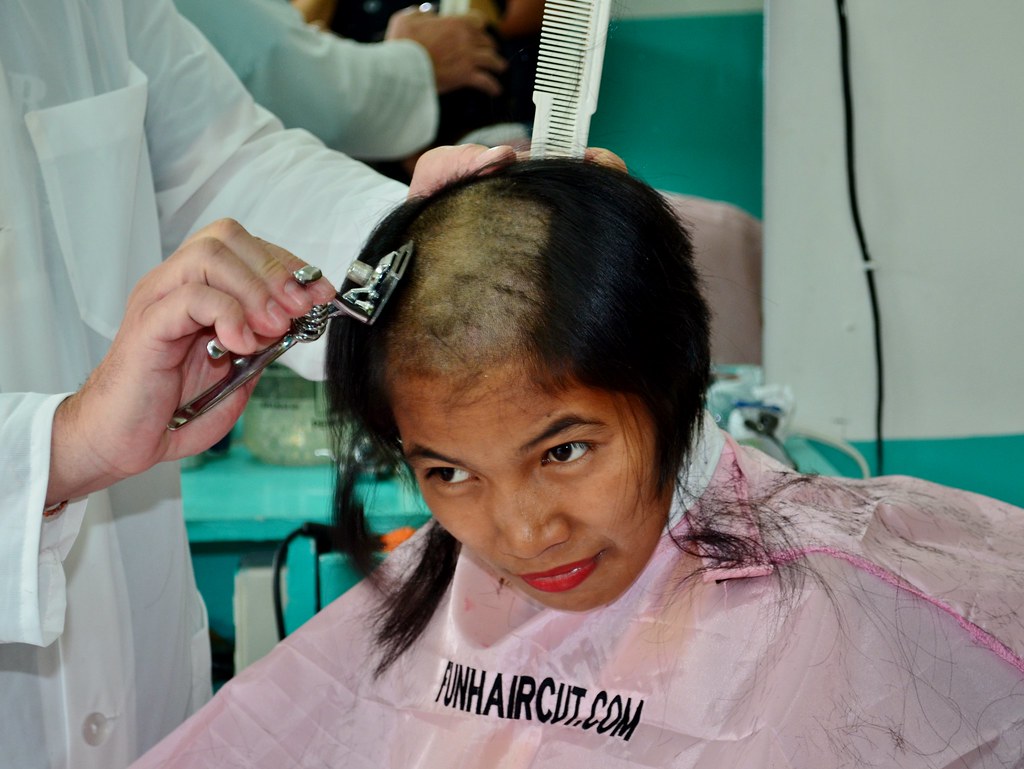In this indoor photograph of a barber shop, an African-American woman is seated in a hairdresser’s chair, wrapped in a light pink cape bearing the words "FunHairCut.com" in black. She has black hair, with some portions already cut, exposing part of her scalp, suggesting she is becoming bald. The barber, a Caucasian man, stands on her left, his face out of the frame, visible only by his white long-sleeve clothing. He holds a trimmer in his right hand and a white comb in his left. The backdrop features a wall with alternating white and green sections, accented by a central mirror reflecting the scene, providing a comprehensive view of the activity. The woman, with striking red lipstick and expressive black eyes, appears focused and slightly pensive. Nearby, the reflection of others seated possibly includes her companions. The image captures a moment of transformation and grooming in a busy barber shop setting.